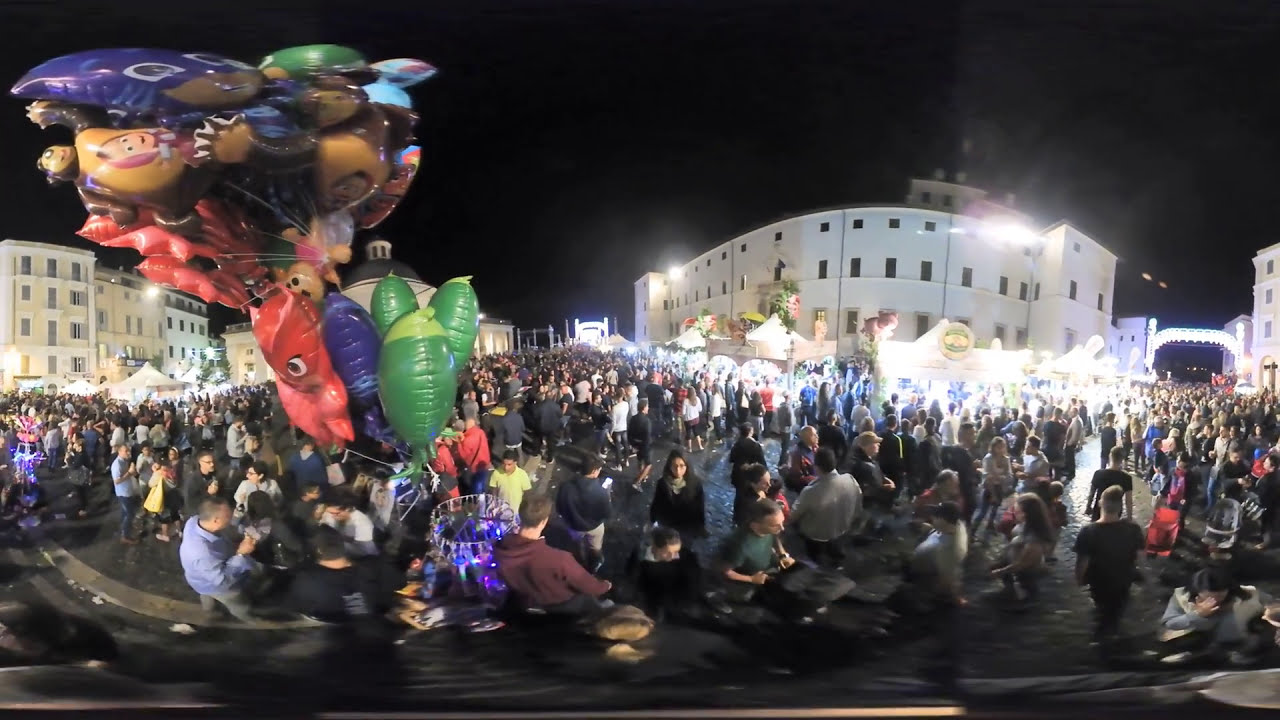The image depicts a bustling nighttime scene in an urban courtyard or city square framed by illuminated white buildings and various light sources. A large crowd of primarily adults, numbering in the hundreds, are either standing or sitting, suggesting an anticipation for an event, possibly a musical performance or festival. The sky overhead is dark, contrasting with the bright lights from the buildings and streetlights, giving the scene a lively yet slightly blurred and distorted appearance, particularly at the bottom.

On the left side of the image, a man is prominently holding an assortment of colorful helium balloons including red, blue, green, and yellow. Among these balloons, one yellow balloon features an animated character resembling a small Caucasian girl with brown hair and eyes, smiling. Other balloons depict multiple characters, possibly from video games, including one that looks like Sonic the Hedgehog.

The far right side of the image shows a white arch, suggesting either an entrance or some architectural feature, helping to frame the scene within the city square. Scattered tents and food stalls are visible along the sides, contributing to the festive atmosphere as people move about. The intricate details and lively elements captured in the image present a vivid portrayal of a vibrant urban nightlife gathering.